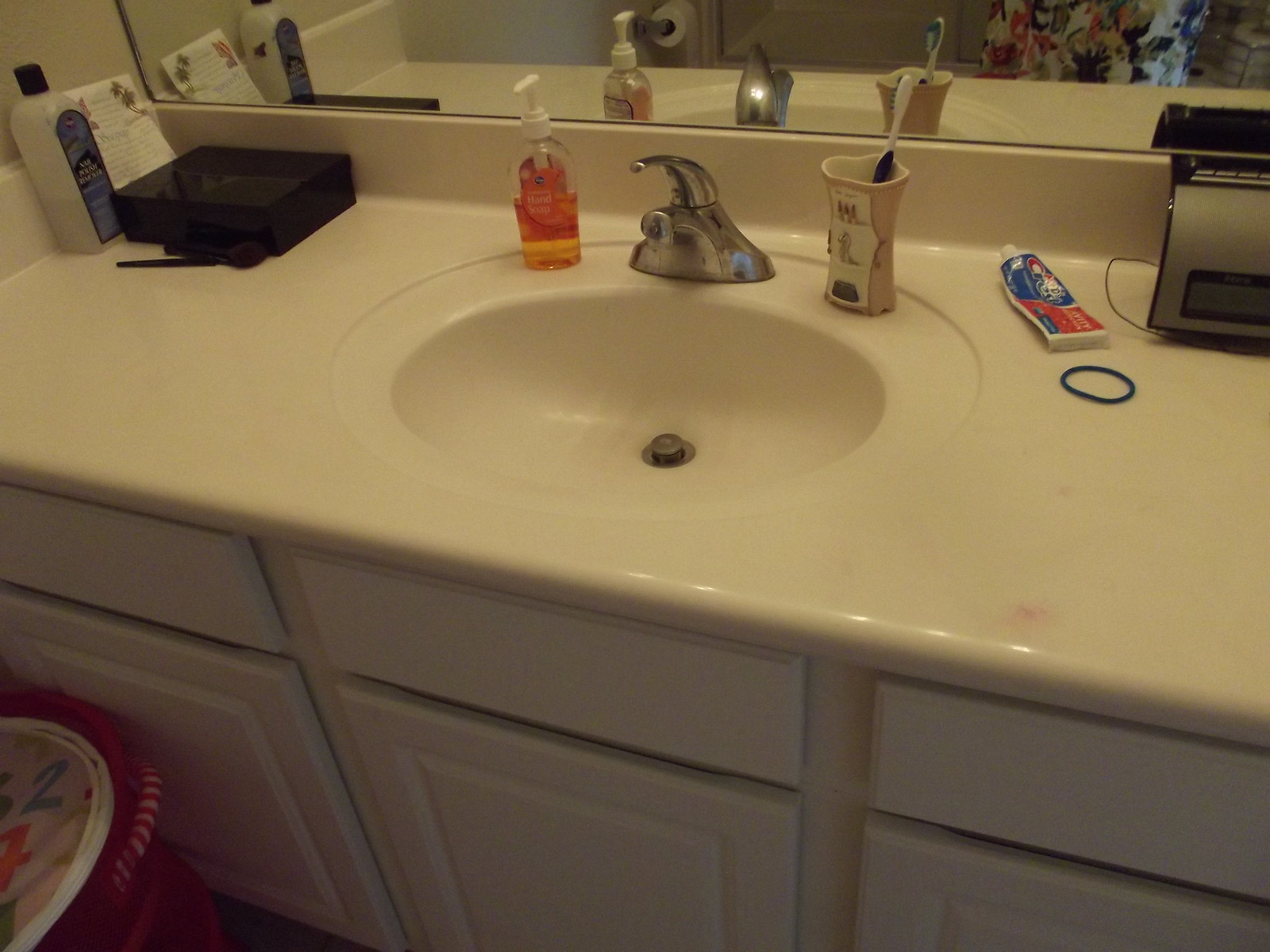In this detailed image of a bathroom, prominent features include a pristine white countertop hosting an oval-shaped basin sink at its center. The sink is equipped with a sleek silver faucet. To the right of the faucet, there's a light brown toothbrush holder adorned with a white design, containing a solitary toothbrush. Adjacent to this holder is a clear bottle filled with orange liquid, featuring a white pump top. On the left side of the countertop lies a shiny black rectangular box, accompanied by a piece of white paper with writing and floral designs. Flanking this setup is a tall, clear plastic bottle containing clear liquid, distinguished by a blue label and a black twist top. Nearby, there is a black blush brush and a black pen-like object resting in front of the black box.

Further to the right of the sink, a white toothpaste tube with a recognizable blue label and red design, likely Crest, can be seen. A blue circular hair tie lies in close proximity to the toothpaste. Against the wall on the right side of the sink, a gray clock with a digital screen adds a modern touch. The background wall is covered by a mirror, capturing reflections of the entire countertop, faucet, orange bottle, toothbrush holder, toothpaste, and clock. The mirror also offers glimpses of a floral-patterned shower curtain and a roll of toilet paper on a wall mount.

Beneath the countertop, three white wooden storage doors provide a neat storage solution. On the floor to the left, a large red laundry basket with a white lid displays a playful pattern of numbers (2, 4, 8), evoking a child-friendly theme.